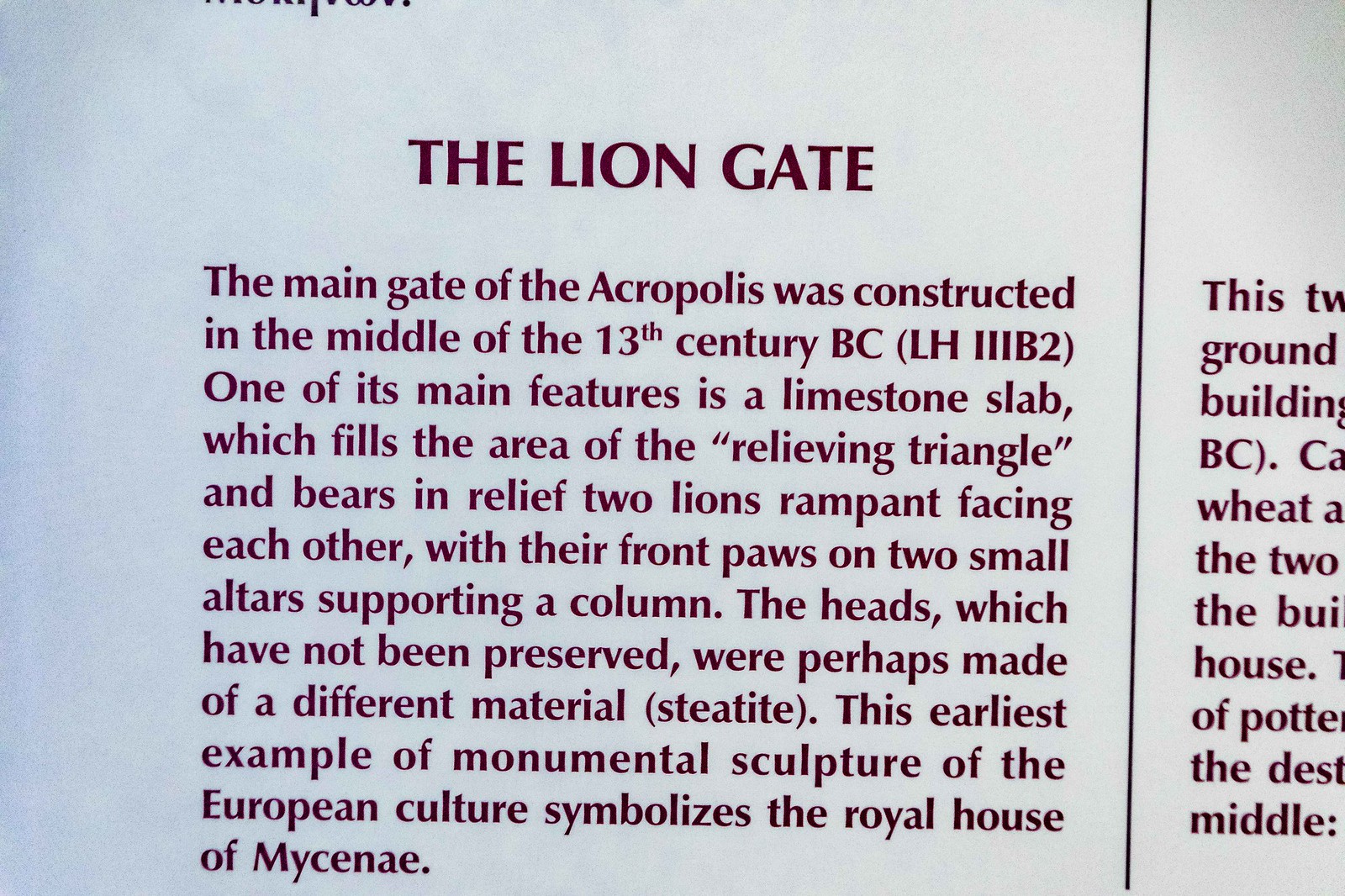The image features an excerpt printed on white paper, detailing the Lion Gate. A black vertical line runs near the right edge of the image, with some partially visible, unreadable text to its right. The main passage, titled "The Lion Gate," is printed in dark font and describes the main gate of the Acropolis, constructed in the 13th century BC (indicated as L-H-I-I-I-B-2). One notable feature of the gate is a limestone slab that fills the area of the relieving triangle. This slab is adorned with a relief of two rampant lions facing each other, their front paws resting on two small altars that support a column. The lions' heads, which likely differed in material such as steatite, have not been preserved. This early example of monumental European sculpture symbolizes the royal house of Mycenae. The text is potentially part of a book or a museum exhibit label, providing rich historical context about the gate.